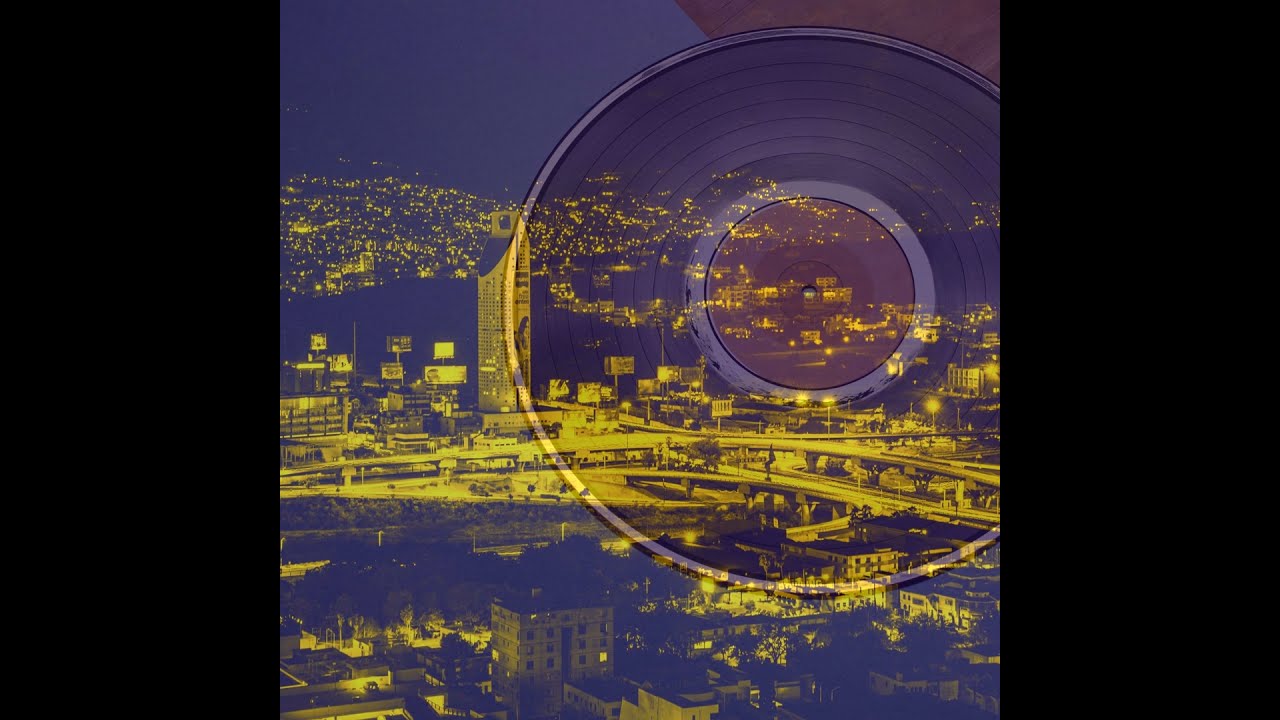The image features a cityscape dominated by a yellow and purple tint, creating a surreal, almost photo-negative look. The urban landscape showcases a network of highways, roadways, and multi-story buildings. Centrally, a tall building or tower block emerges amidst the intricate web of roads and lights. In the distance, a hill lit by numerous lights stretches across from left to right, framing the city. The city extends into the foreground with trees and additional buildings, yielding a comprehensive view of the metropolis.

Overlaid on the upper right portion of the image is a semi-transparent vinyl record, featuring black grooves and a red (some say brown) center. The record occupies a significant portion of the image, roughly three-fifths of the space, yet remains translucent enough to allow the cityscape to be visible beneath it. The image is framed by a thick border on the left and right sides, but the top and bottom are borderless. Overall, the striking color palette and the overlay of the record suggest a creative, possibly album cover-like design, though no text is present.